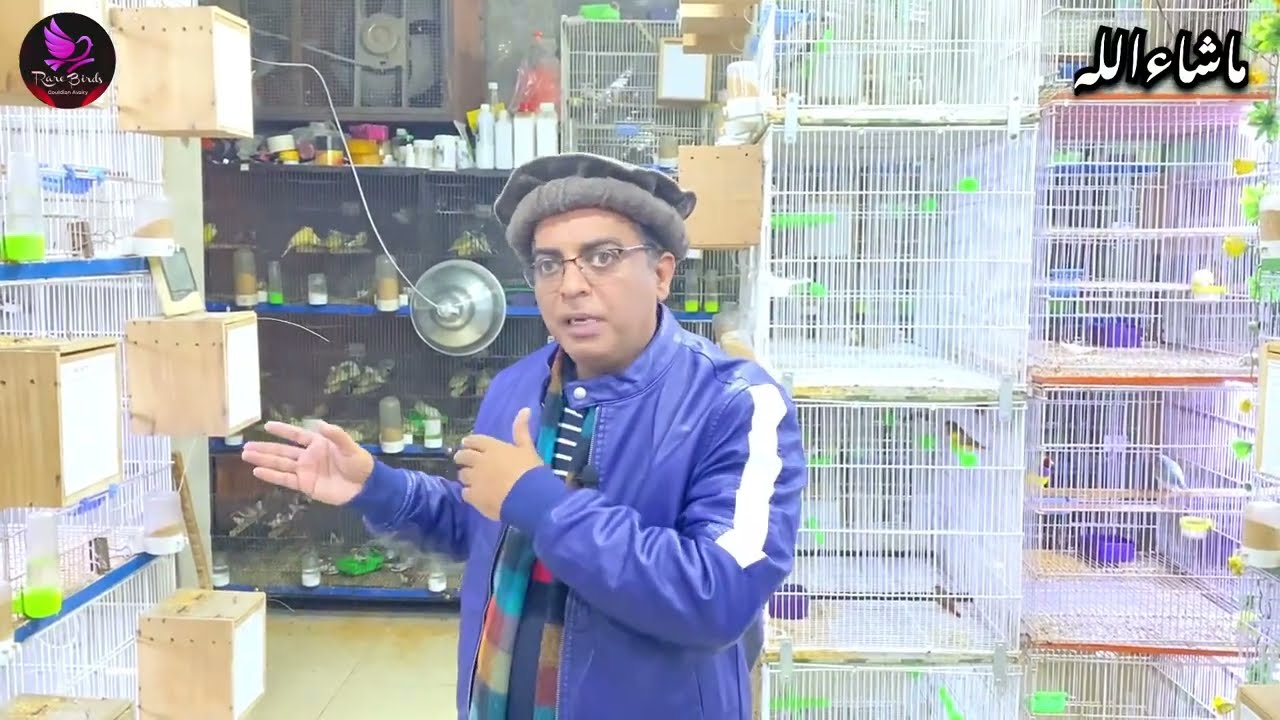The image features an Indian man in a vibrant blue leather jacket with a white stripe down the sleeves and a distinctive gray knit hat. He wears glasses and stands behind a plexiglass window, which has a mouthpiece for speaking. The man appears to be explaining or showcasing something as he gestures with his hands raised towards an array of white wire bird cages. While the cages directly in front have fewer birds, there are more cages and a noticeable number of parakeets of various colors in the background. In addition, small wooden boxes are visible in front of some of the cages. The scene suggests that this location is a pet store specializing in birds. In the top right corner, text in an Indian language further grounds the setting culturally and linguistically.